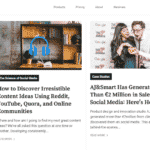Caption:

"A dark and somewhat gloomy, pixelated image captures the top portions of two overlapping blog posts. In the upper left corner, an image of a bookshelf, which also doubles as a desk, sets a somber tone. In front of the bookshelf, a blue headphone icon is noticeable. The visible text of the first blog post's title reads, 'How to Discover Irresistible Content Ideas Using Reddit, YouTube, Quora, and Online Communities.' To the right side of the image, a man and a woman are seen touching hands in front of what appears to be an awards ceremony backdrop. The partial title of the second blog post reads, 'Smart ... Two Million in Sales, Social Media, Here’s...,' with several lines of highly pixelated text below it."